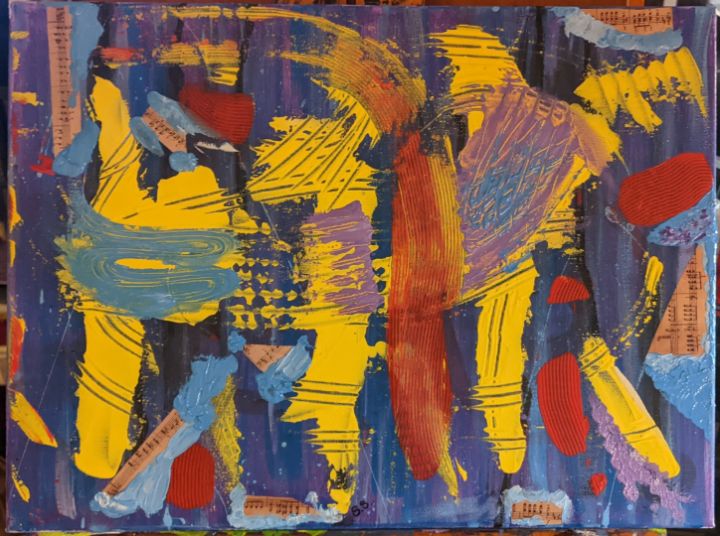This rectangular painting, measuring approximately 5 inches wide by 4 inches high, features an abstract design with a very thin 1/8 inch border. The primary background consists of deep purples and blacks, enhanced with splashes of various blues. Dominating the composition are three large, vertical stripes of gold or yellow, possibly suggesting humanoid figures, which traverse the painting from left to right. Nestled between the second and third of these figures is a bold red-orange swipe of paint that stands out dramatically. 

From left to right, a wide horizontal stripe transitions smoothly from blue to purple, lending a dynamic flow to the artwork. Encircling these elements are numerous red stripes and dots, adding intricate details. The painting also incorporates unique textures, with orange paper embedded into the paint, some featuring what appear to be black music notes. The overall effect is a vibrant, mesmerizing array of yellow, purple, red, orange, blue, black, and brown, creating a striking and colorful abstract scene.